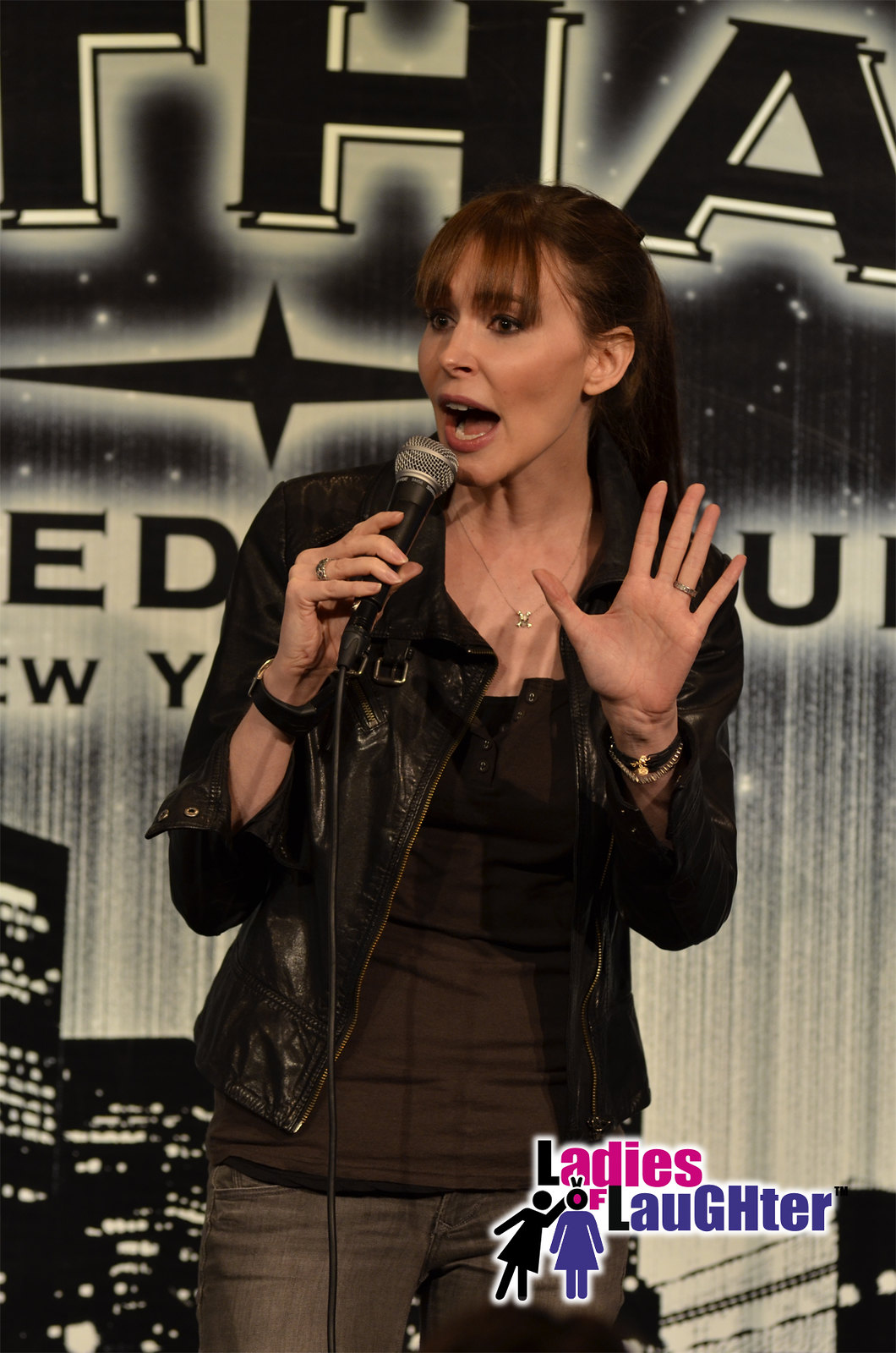This detailed photograph captures a female comedian performing on stage, bathed in the monochromatic ambiance of a black and white cityscape backdrop that resembles New York City. The stage displays various words obscured by her presence, yet distinctly features the "Ladies of Laughter" logo at the bottom right-hand corner, comprising black and purple outlines of two women in skirts with one pointing at the other's head.

The comedian, a white woman with brown eyes and straight, reddish-brown hair pulled back into a ponytail, has bangs that graze her eyebrows. Her expressive face adorned with makeup, including lipstick and eyeliner, showcases a large smile as she holds a microphone close to her mouth, mid-speech. Her left hand is raised at shoulder level in a gesture akin to a stop signal. 

She dons a dark leather jacket—described variably as black and chocolate brown—over a brown shirt, paired with dark-colored jeans. Accessorized with a silver necklace, bracelets, rings, and a watch, her ensemble reflects a blend of casual and chic. The backdrop cannot be fully deciphered due to her positioning, but it complements the comedic and lively atmosphere of her stand-up performance.